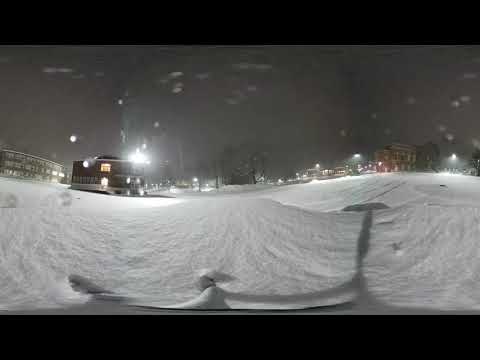In this nighttime footage of a cold, snowy scene, the surroundings are almost eerily quiet with no visible people present. Snow is blanketing the ground and falling gently from the dark sky, creating a serene winter atmosphere. The camera, likely positioned on a street lamp or a tall structure, such as a building, captures a wide view, possibly overlooking a schoolyard or a field.

The left side of the image reveals a large, three-story brown building with many windows, some of which are brightly illuminated, suggesting occupancy. Adjacent to it is a slightly smaller, two-story structure that stands out with a bright white light. On the right side, there's another significant dark brown building resembling a school, made from brickwork.

The scene is illuminated by artificial lights, likely street lamps, casting a soft glow against the snow-covered landscape. This small town scene is full of contrasting shades of white, black, and various grays, heightening the tranquility and simplicity of the snowy night.